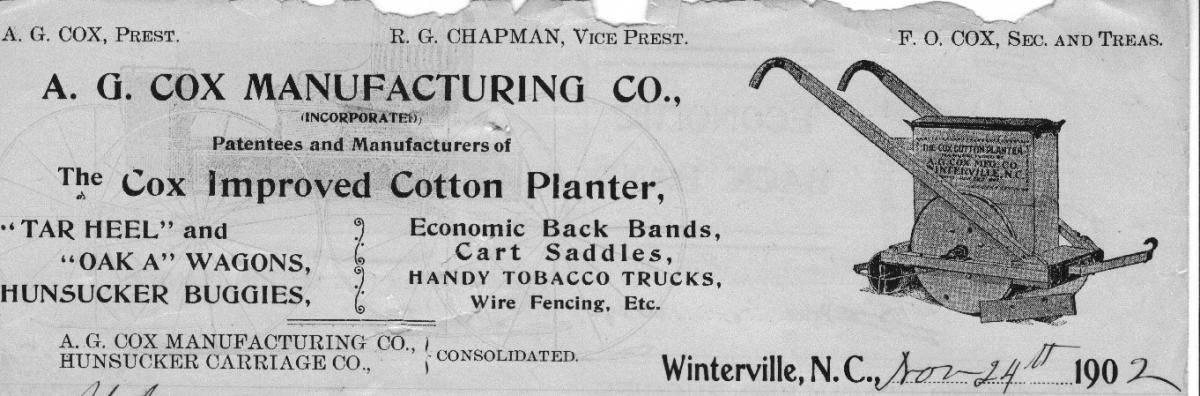This image depicts a weathered and torn gray piece of paper resembling an old receipt or advertisement. At the top left corner, it states "A.G. Cox Pressed," followed by "R.G. Chapman Vice Pressed" in the center, and "F.A.O. Cox Sec and Treas" (Secretary and Treasurer) in the top right. Below these titles, in prominent black font, reads "A.G. Cox Manufacturing Company, Incorporated."

The document further details the company's products, listing "Patentees and Manufacturers of the Cox Improved Cotton Planter, Tarheel and OK Wagons, Hunsucker Buggies, Economic Backbands, Cart Saddles, Handy Tobacco Trucks, Wire Fencing, etc." On the left side, "Tarheel and OK Wagons" and "Hunsucker Buggies" are separately mentioned. Centrally displayed are "Economic Backbands, Cart Saddles, Handy Tobacco Trucks, Wire Fencing, etc."

At the bottom-left corner, the paper consolidates "A.G. Cox Manufacturing Company" with "Hunsucker Carriage Company." The bottom right corner specifies the location and date as "Winterville, North Carolina, November 24, 1902." Additionally, there is an illustration of a cotton planter featuring handles, wheels, and a central vertical rectangular box, symbolizing the craftsmanship touted by the company.